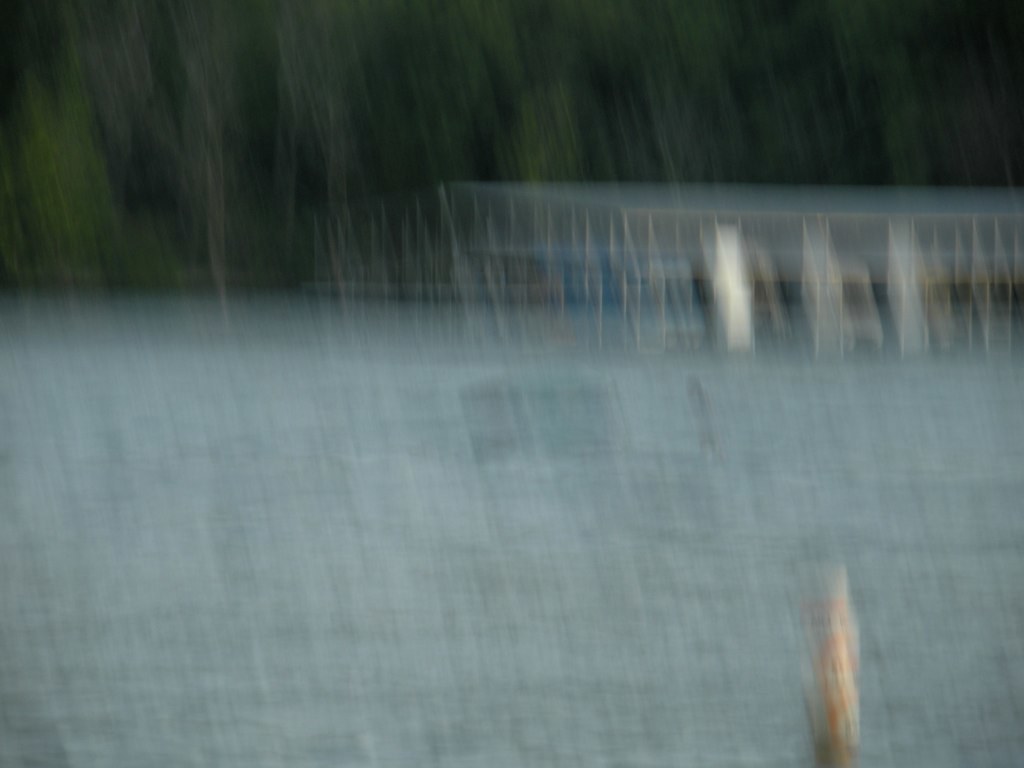This extremely blurry and pixelated nighttime photograph predominantly features a bluish-green lower section, possibly indicative of water. The center left showcases a row of indistinct trees that stretch horizontally across the image. In the lower right corner, a light brown wooden fence post stands out. The upper third of the image contains shadowy tree trunks, with minimal detail extending into the background. A white or light tan structure with many poles, perhaps a dock or slanted roof, occupies about a third of the way down on the right side. The entirety of the photograph is marred by out-of-focus vertical lines, enhancing the ghostly, nauseating appearance described by the viewers. Main visible colors include green, blue, white, and brown.